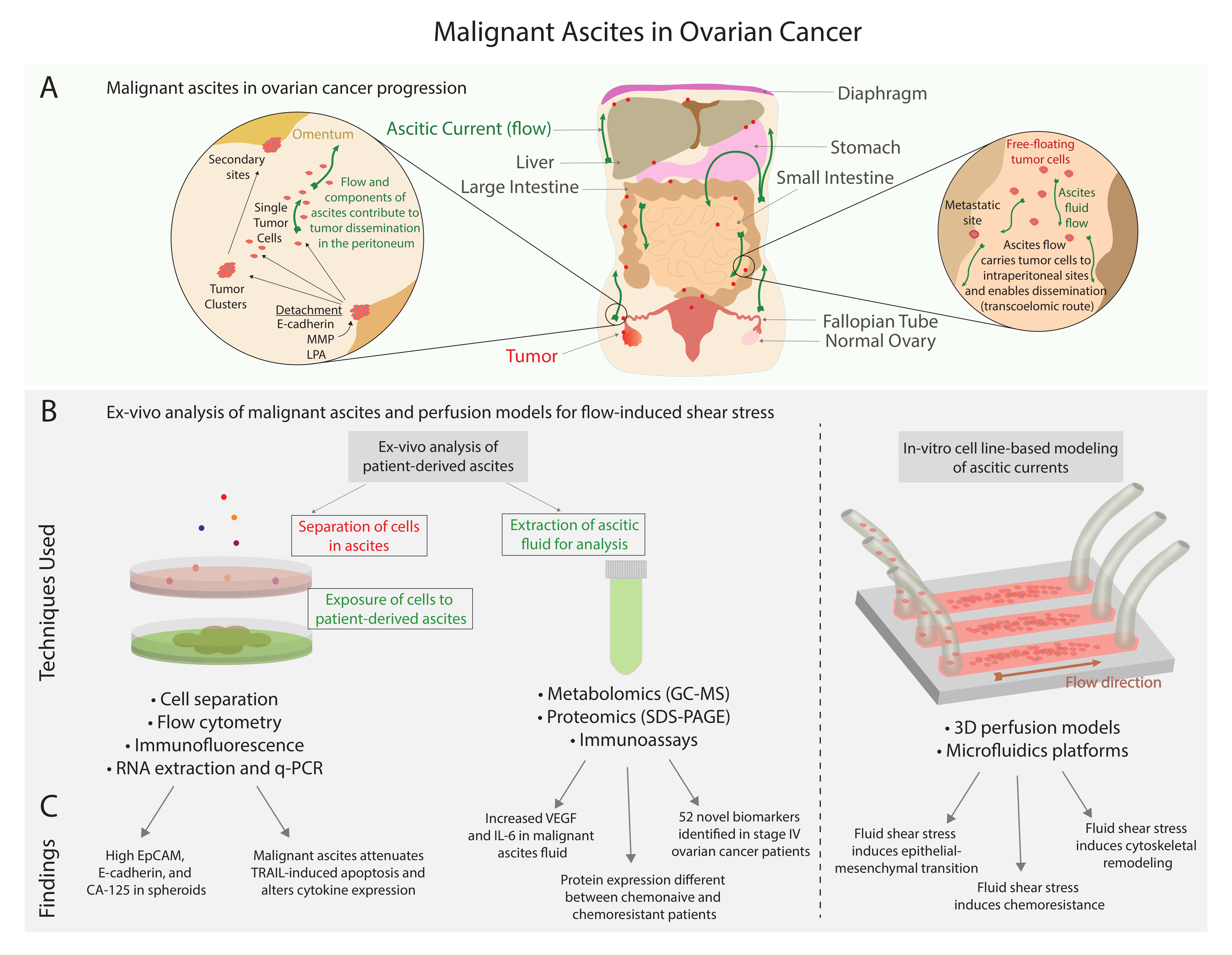The detailed illustration titled "Malignant Ascites in Ovarian Cancer" is divided into three sections, A, B, and C. Section A depicts the anatomical area affected by ovarian cancer, showcasing a detailed view of the abdomen, including the liver, diaphragm, stomach, large intestine, and small intestine. It highlights the role of malignant ascites in the progression and dissemination of ovarian cancer, revealing how ascitic fluid flow facilitates the spread of tumor cells to intraperitoneal sites. Magnified images also illustrate single floating tumor cells, tumor clusters, and molecular components like E-cadherin and PLPA.

Section B focuses on ex vivo analysis of malignant ascites, presenting a perfusion model to examine flow-induced shear stress. It illustrates processes such as the separation of cells in ascitic fluid, represented in a petri dish, and the extrusion of fluid for analytical purposes. Techniques like flow cytometry, immunofluorescence, RNA extraction, and qPCR are detailed to demonstrate how these methods contribute to understanding cancer cell behavior.

Section C delves into in vitro saline-based modeling of ascitic currents, showing fluid flow direction with a detailed depiction of tubes and the effects of fluid shear stress. This section underscores the importance of fluid dynamics in cancer research, emphasizing how these processes can attenuate stress-induced apoptosis in tumor cells.

Overall, the illustration integrates anatomical, molecular, and analytical perspectives to provide a comprehensive overview of the mechanisms and experimental approaches related to malignant ascites in ovarian cancer.